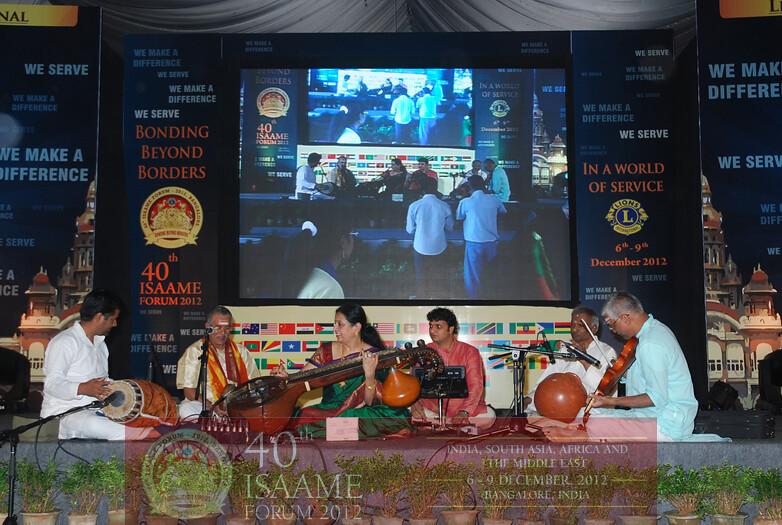This vivid photograph captures the lively atmosphere of the "40th ISAAME Forum 2012" held in Bangalore, India, on December 9, 2012. The event title, "Bonding Beyond Borders," is prominently displayed on gray curtains flanking a large video screen that replicates the on-stage activities, including audience reactions and other festivities. The stage itself is dotted with lush green plants in reddish-brown flower pots atop a gray floor, adding a natural touch to the vibrant scene.

At the forefront, a five-member musical band is in mid-performance. The band is arranged from left to right: A musician in an all-white outfit plays a pair of bongo drums, next to a woman in a green, red, and blue dress, adorned with a purple hue, delicately plucking a brown sitar. Beside her sits an older gentleman, draped in white with a colorful red, yellow, and orange scarf, vocalizing into a black microphone. To his right, another man in a red shirt and white pants is engaged in his musical endeavor. Completing the lineup is a violinist in an all-white outfit, playing his brown instrument with poised concentration.

In the background, above the screen, the text "Bonding Beyond Borders" and "We Serve, We Make a Difference" encapsulate the philanthropic spirit of the gathering, with additional details highlighting the event’s international scope, mentioning South Asia, Africa, and the Middle East.

The musicians' attire adds splashes of color against the blue background of the video display, with shades of white, pink, and green standing out. Meanwhile, three individuals standing before the stage, attired in white shirts and blue jeans or pants, contribute to the celebratory ambiance. The black microphones and the brownish instruments add to the intricate tableau, making it an engaging piece that evokes the sounds and sights of a festive musical celebration centered around unity and service.